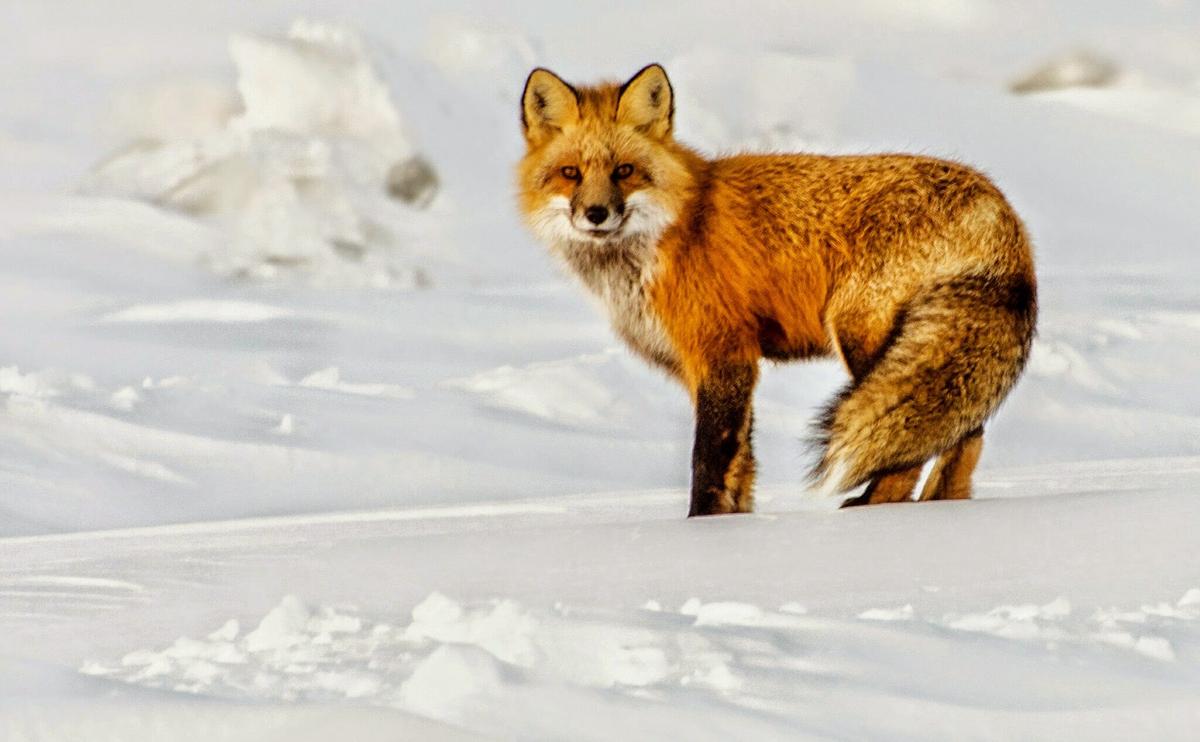The close-up photograph captures a lone fox standing still in a snowy landscape, seemingly posing for the camera. The snow-covered background is slightly hilly but otherwise unaltered, emphasizing the fox as the main subject. Bathed in daylight, which casts subtle shading on the snow, the fox gazes directly at the photographer with ears perked up and eyes fixed on the lens. The fox's rich winter coat is detailed and varied: the lower half of its face is white, transitioning to darker fur around the eyes and a reddish-umber body. Its legs show a blend of black, while its bushy tail is a mixture of tans, browns, and blacks. Tracks in the snow hint at movement, but the fox remains the focal point, its vivid coloring and attentive stance drawing immediate attention. The bright, snow-muted background enhances the sharpness and detail of this magnificent creature, highlighting its seasonal adaptation with a thicker, fluffier coat.